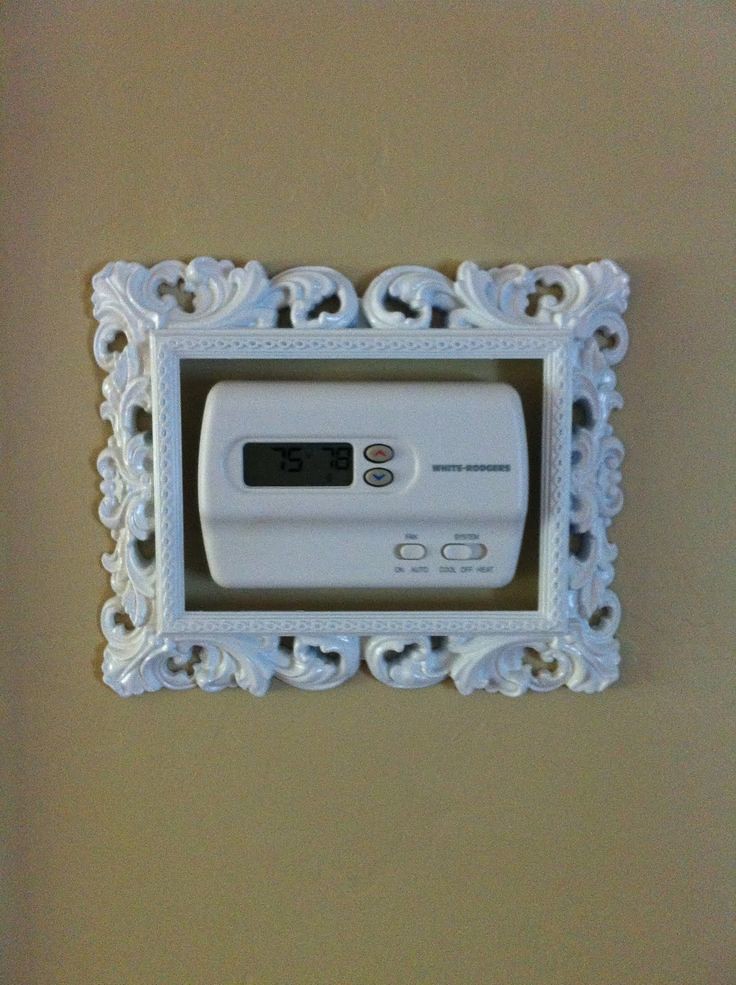A blurry photograph showcases an outdated White Rodgers plastic thermostat mounted on a light brown or khaki-colored wall. The rectangular thermostat features a very small, old-style LCD display, which is difficult to read due to its low contrast. Adjacent to the display are two buttons, one with a red up arrow and the other with a blue down arrow. At the bottom of the thermostat are two white buttons, although their labels are not clearly discernible. Surrounding the thermostat is a decorative white frame designed to resemble wrought iron, adding an ornamental touch to an otherwise functional piece of equipment. The thermostat has a switch with labels like "Cool," "Off," and "Heat," as well as another label reading "On" and what seems to be "Auto" for the fan, though these details are hard to confirm due to the photograph's poor focus.